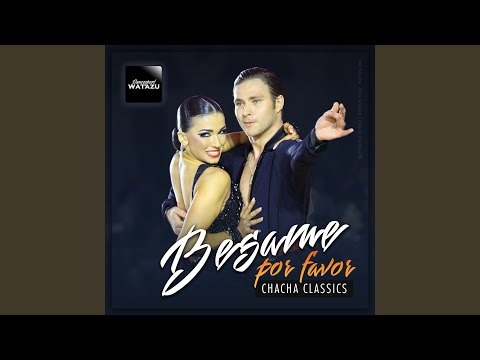The image appears to be an advertisement or an album cover, possibly for a Spanish-themed dance collection titled "Bésame Por Favor Cha Cha Classics." It features a dancing couple against a black background, framed by horizontal black bands at the top and bottom. The man, positioned on the right, has fair skin and slicked-back dark black hair. He is wearing a long black shirt or dance suit, and his right arm extends outward with his pinky finger out and middle finger slightly curled. His left arm is around the woman's back. The woman, standing chest-to-chest with the man on the left, has brown skin and her black hair pulled tightly into a bun. She is adorned with bright lipstick and wears a sleeveless, backless black dress with white dots across the chest. Her left arm is around the man's neck, and her right hand rests on his chest. The top left corner of the image contains white text within a black box, which is somewhat unreadable but possibly says "Huatazi." Also featured in white cursive writing is "Bésame," followed by "Por Favor" in orange, and finally "Cha Cha Classics" in white.